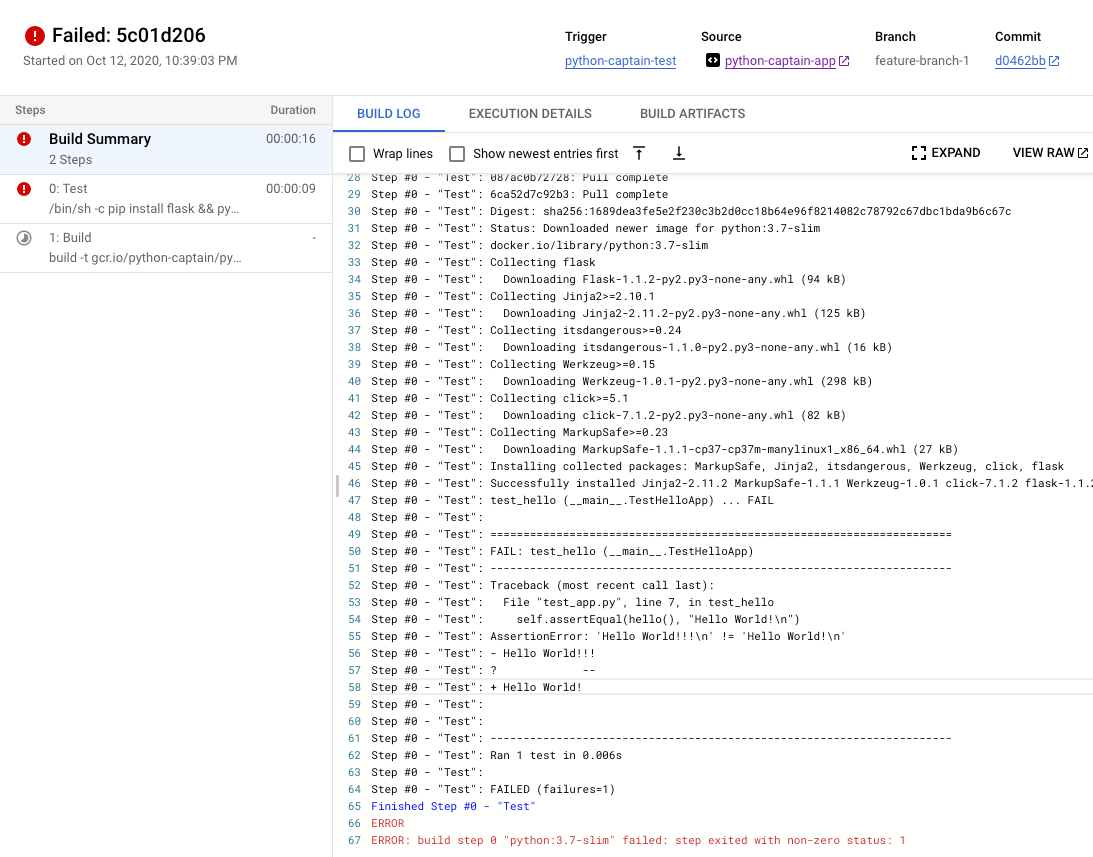The image depicts a website layout with a clean white background. 

- In the upper-left corner, there's a prominent red circle featuring a white exclamation point inside it. 
- Adjacent to this icon, the word "FAILED" is displayed in bold, black print, followed by a colon. 
- The subsequent text reads "c01d206," all in lowercase.
- Below this, it states "Started on October 12th, 2020, 10:39:03 PM."

Moving towards the center and the right side of the page:
- There are entries for "trigger," "source," "branch," and "commit."
- "trigger: Python_caption_test"
- "source: Python_captain_app"
- "branch: feature_branch_1"
- "commit: d0462bb"

On the left-hand side of a banner:
- The title "STEPS" is displayed, while "DURATION" is indicated on the right.
- Three steps are listed below:
  1. Build Summary (2 steps) - marked with a red circle and white exclamation point.
  2. Test (0 tests) - marked similarly.
  3. Build (1 build)

Additionally, underlined in blue and written in capital letters, the terms "Build Log," "Execution Details," and "Build Artifacts" are presented.